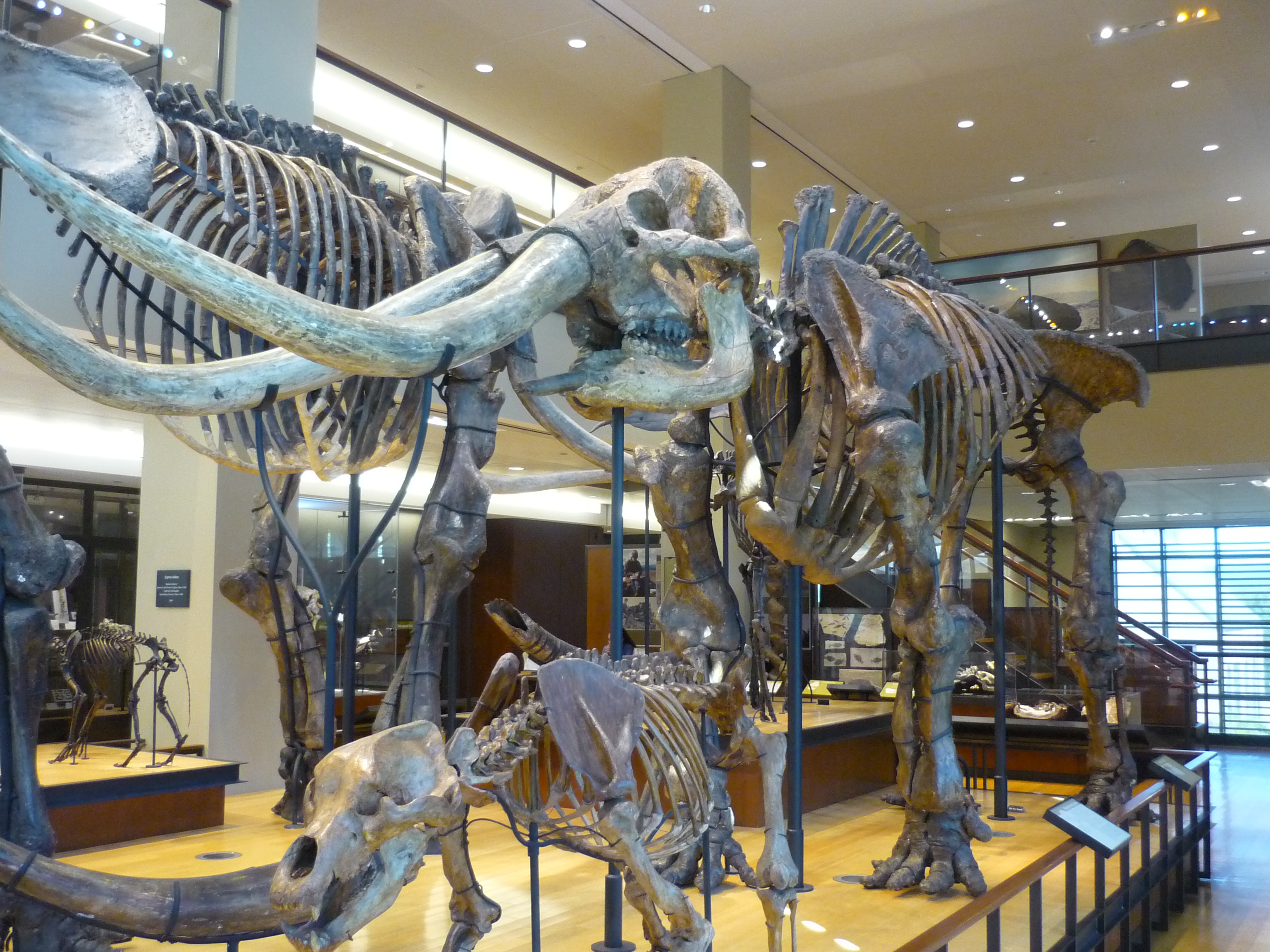The image depicts a large, well-lit science museum display featuring the assembled bones of prehistoric animals. Dominating the scene is the towering skeleton of an extinct elephant-like creature, possibly a mastodon, with two massive tusks curving outward from its prominent skull. This impressive skeleton, standing around 10 to 12 feet tall, is meticulously put together, showcasing its large leg bones and a skeletal structure that spans almost the entire height of the display area. 

In front of this large specimen is a smaller, likely juvenile skeleton, devoid of tusks but featuring a proportionally long skull and small spinal spikes. Despite its diminutive size, this skeleton mirrors the larger one in form. Both are positioned on a polished yellow wooden platform surrounded by a small railing, which demarcates the exhibit.

Further in the background stands another even taller skeleton, though only its towering body is visible as the head remains out of the frame. This third skeleton looms over the display, adding to the grandeur of the scene.

The setting itself is expansive, with a gray and yellowish-brown ceiling supported by white columns housing various pot lights. These lights effectively illuminate the entirety of the scene. A visible staircase and a large window with open blinds allow additional light to filter in, creating a bright and inviting atmosphere. An upper level with a glass railing encircles the exhibit, providing an elevated vantage point for visitors to peer down at the ancient relics below.